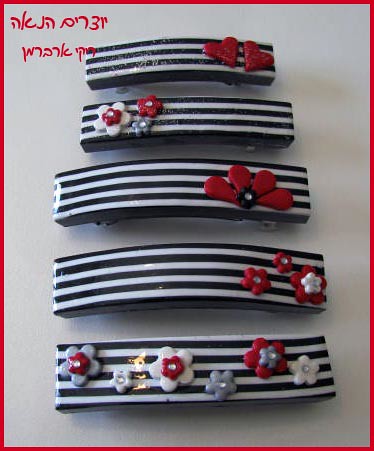The image depicts a collection of five rectangular hair clips arranged vertically against a gray background with a thin red border. Each hair clip features a consistent black and white striped pattern as a base and varying decorative elements. The top hair clip, predominantly plastic, has two red heart-shaped plastic emblems on the right end. The second clip below it showcases three flowers on the left: a white petaled flower with a red center and clear stone, a smaller red flower with a clear stone, and a blue flower with a clear stone. The third clip has a red flower with four petals and a shiny silver center on the right. Moving down, the fourth clip displays three red flowers on the right, with the largest one having a prominent white center. The bottom clip features an assortment of flowers in red, white, and gray colors, each adorned with a clear stone in the center. The hair clips appear to be made of plastic, and part of the barrette clip mechanism is visible beneath the decorations. Additionally, there is an inscription in an unidentified oriental script in red at the top of the image.